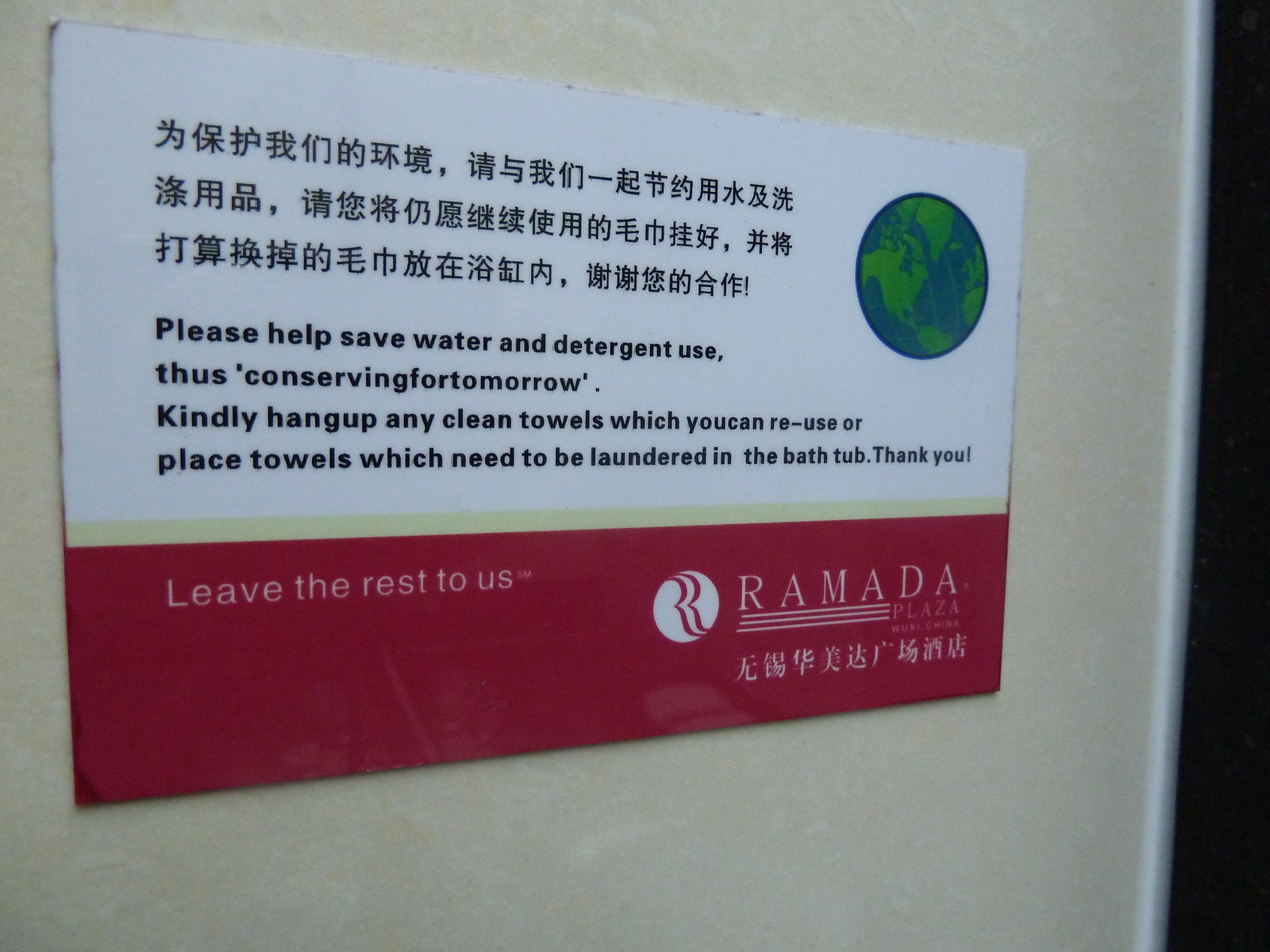The photograph showcases a rectangular plaque mounted on a beige-colored wall next to a black doorway. The plaque is divided into several sections. At the top, there are three lines of foreign characters, potentially Chinese or Japanese. Below this, there is a section with black sans-serif text on a white background that reads: "Please help save water and detergent use, thus conserving for tomorrow. Kindly hang up any clean towels which you can reuse or place towels which need to be laundered in the bathtub. Thank you." On the top right corner of this section, there is a graphic of the Earth showing the Americas and parts of Europe and the oceans painted blue. At the bottom of the plaque, there is a red bar with the white text, "Leave the rest to us." Next to this text is the Ramada Plaza logo, which consists of a cropped white circle with an outlined letter "R" in white, followed by more foreign characters. The plaque combines both informative and promotional elements in an organized layout.